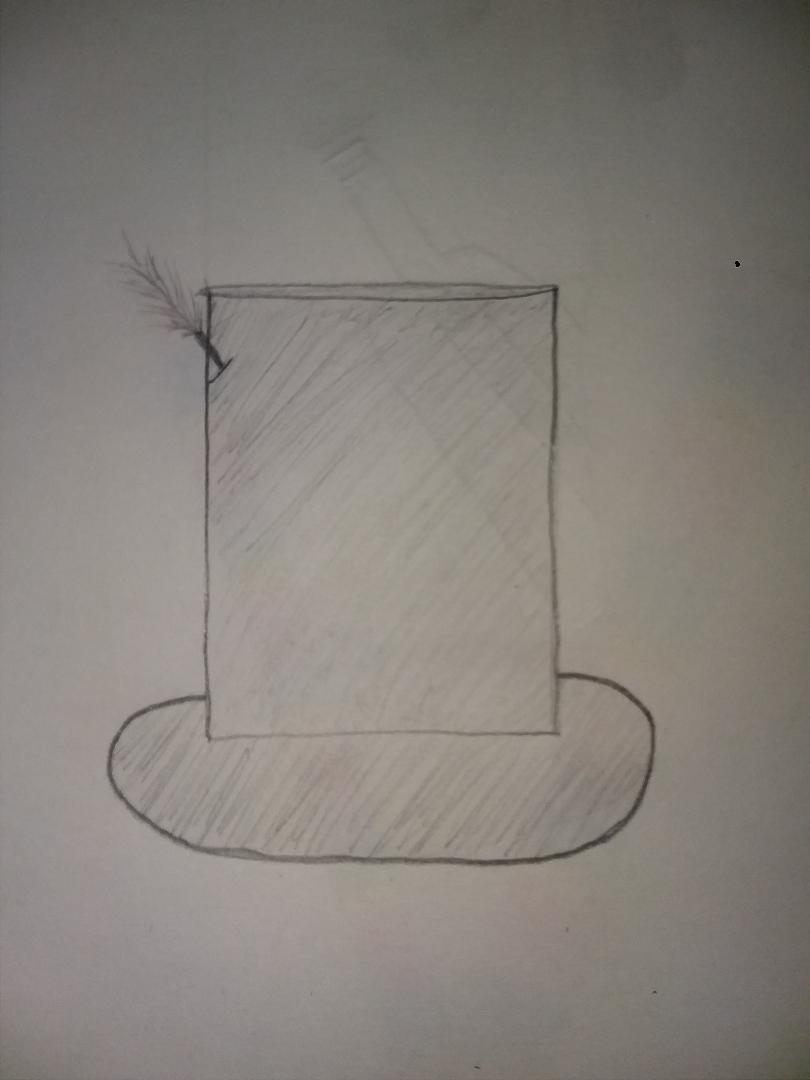The image features a meticulously hand-drawn black and white sketch on a pristine white sheet of paper. At the center of the composition lies an intricate object, primarily composed of two distinct shapes: a square at the top and an oval platform below it. The square and oval elements are meticulously shaded with pencil, giving them a textured, three-dimensional appearance. Protruding from the top left corner of the square is a curious detail resembling a firecracker, adding an intriguing focal point to the drawing. This finely detailed illustration highlights the artist's skillful use of shading and form, creating a captivating piece of black and white artistry.